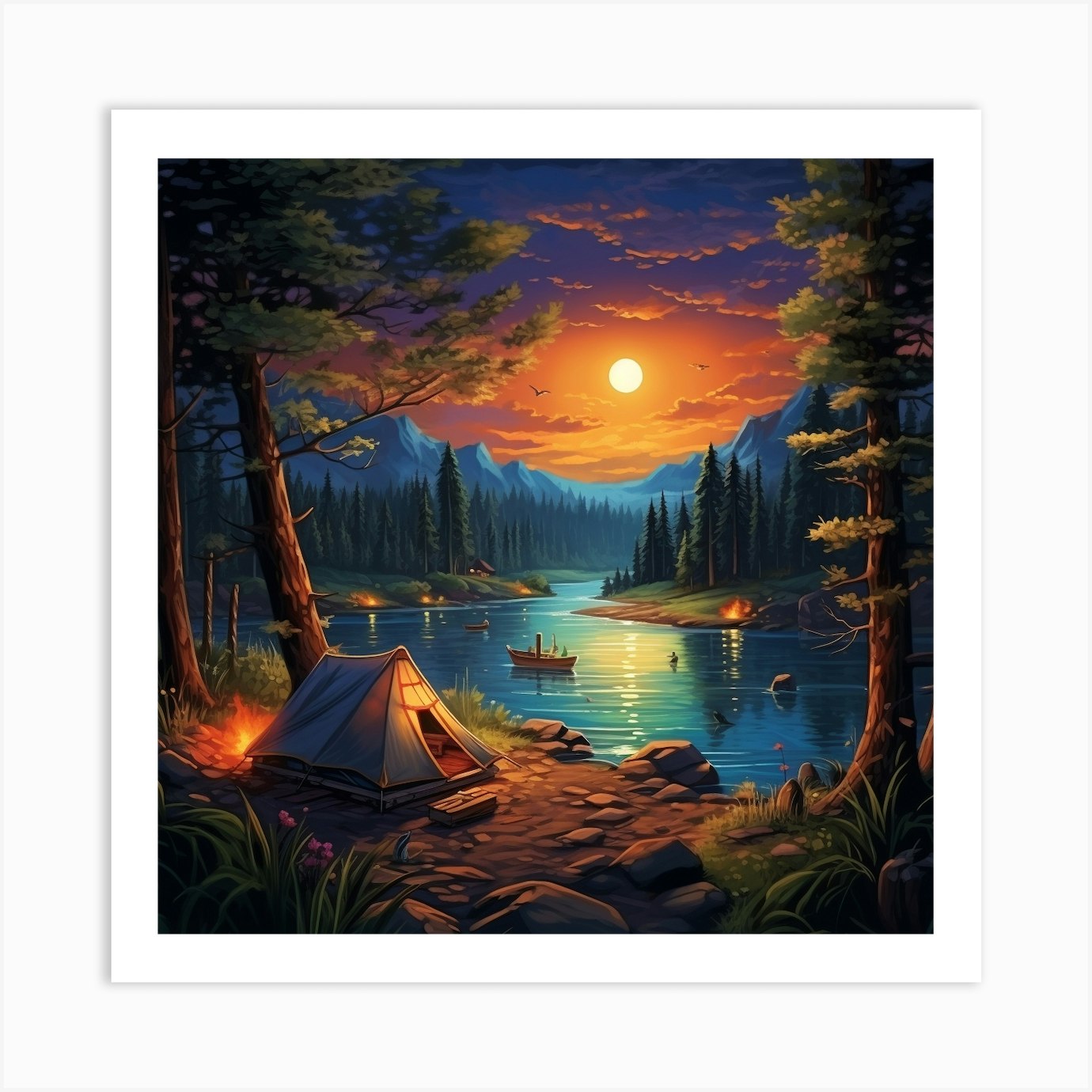The hand-drawn painting, encased in a thick white mat, depicts a serene, nature-themed campsite nestled next to a lake winding through a majestic mountain range. Central to the scene is a small white fabric tent, bathed in a warm orange light, resting on a rocky surface near the water's edge. Flanking the tent are trees that stretch from one side of the painting to the other. A campfire glows softly to the right across the water, near another tent. The tranquil lake, reflecting the moon's light, is home to a canoe floating gently on its surface. In the backdrop, the lake shimmers as it meanders, surrounded by an array of campfires and tents that dot the orange-lit shoreline. The sky, adorned with clouds, transitions from a deep orange to purple, indicating a vibrant sunset or twilight, with a prominent full moon illuminating the scene. The distant mountain range glows with blue hues, while a thick line of trees marks the base, creating a captivating contrast between the natural elements. Scattered supplies in front of the main tent and occasional flowers add a touch of detail to the rocky campsite, enriching the overall composition of this idyllic wilderness retreat.